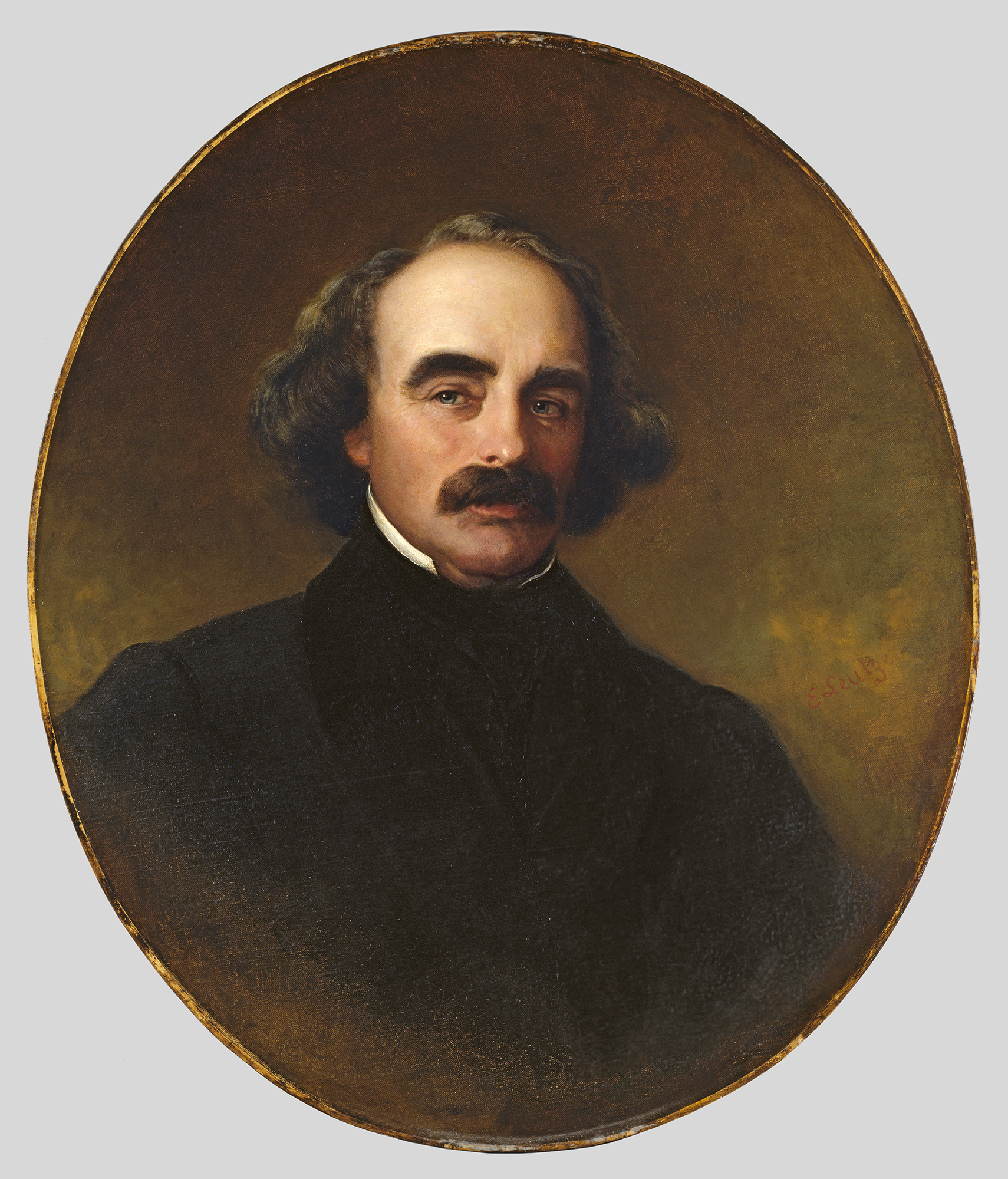This image appears to be an old-style watercolor illustration of a distinguished elderly white man with a prominent, thick mustache and no beard. His hair is a mix of grey and black, long enough to curl around his ears, giving it an Einstein-like appearance, though he has a balding spot at the front. The man's eyes are a captivating shade of green or blue, and he is donned in a black suit with a white shirt peeking from beneath a black undershirt. The background is a blend of light and dark brown with a hint of yellow on the right side, surrounded by a light grey circular backdrop. His contemplative expression suggests he might be lost in thought or gazing at something out of view. The blend of colors and shadow effects gives the image a nostalgic, almost timeless feel, reminiscent of the 1800s or early 1900s.